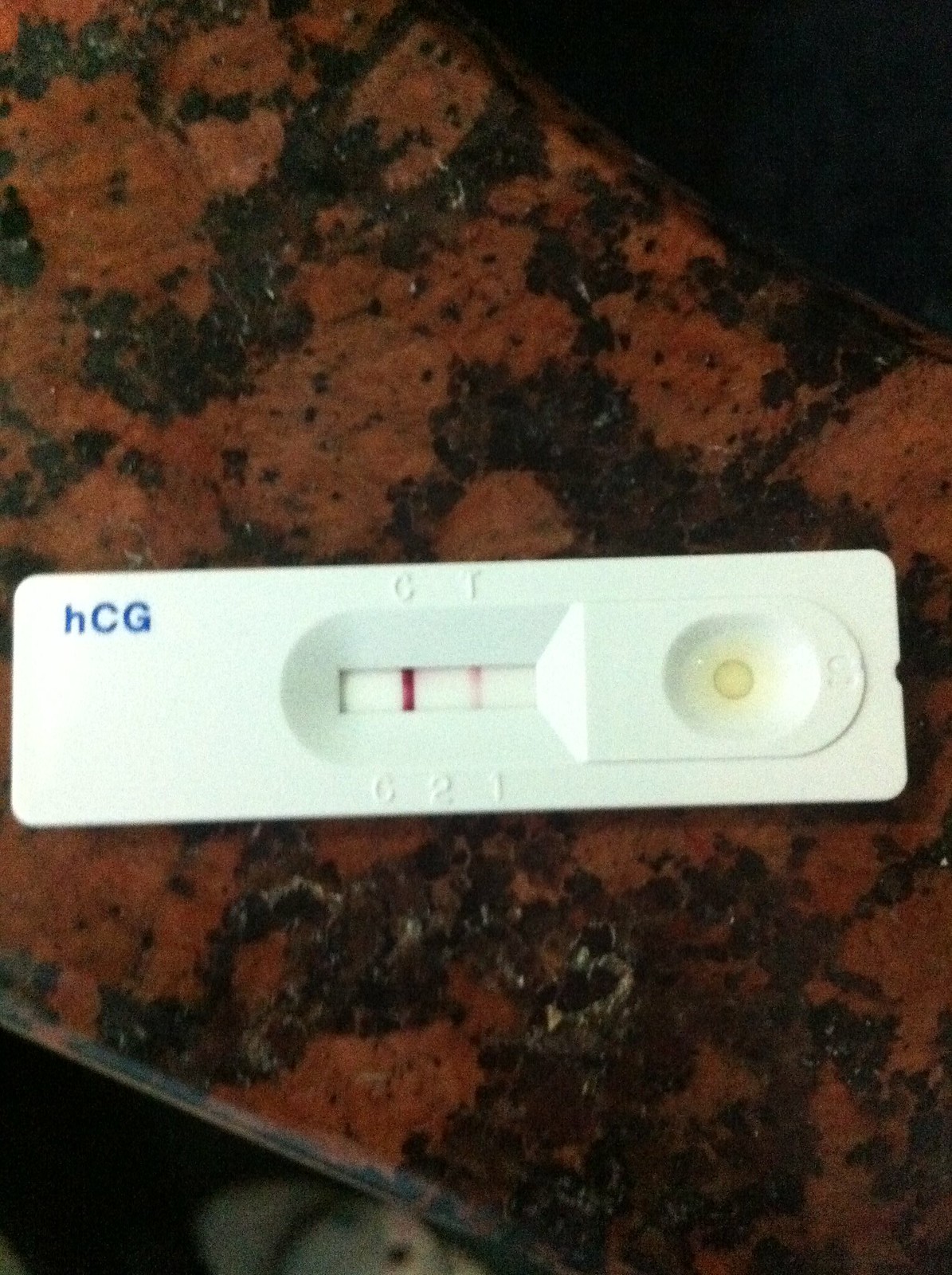An up-close image captures a COVID-19 test indicating a positive result, prominently placed on a brown and black countertop, which appears to be made of epoxy-covered cork. The detailed texture and patterns of the countertop provide a striking contrast to the stark appearance of the test device, emphasizing the significance of the positive outcome. This test outcome confirms that the individual to whom it belongs has contracted COVID-19.